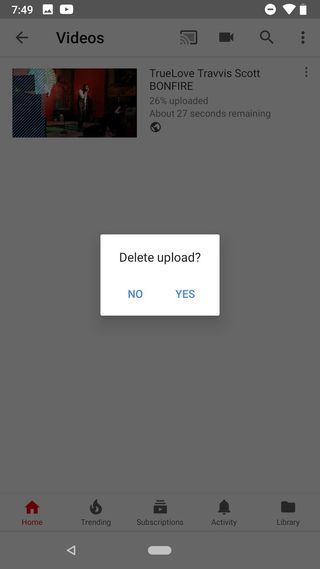This screenshot, captured from a mobile phone, showcases the YouTube application interface. The top of the screen displays typical mobile indicators: on the left, the current time is followed by a camera app icon and the YouTube app icon. On the right side, it shows a minus symbol icon, a Wi-Fi signal indicator, and a battery level icon.

The main content of the screenshot reveals a user's video upload progress within the YouTube app. The user has uploaded a single video titled "True Love Travis Scott Bonfire," which is currently 26% uploaded, with approximately 27 seconds remaining until completion. However, the entire upload interface is dimmed out due to an overlaying pop-up box centered on the screen.

The pop-up box, stark white for emphasis, poses the question "Delete upload?" There are two options at the bottom of this dialog box: "No" on the lower left and "Yes" on the lower right, allowing the user to confirm or cancel the deletion of the video upload.